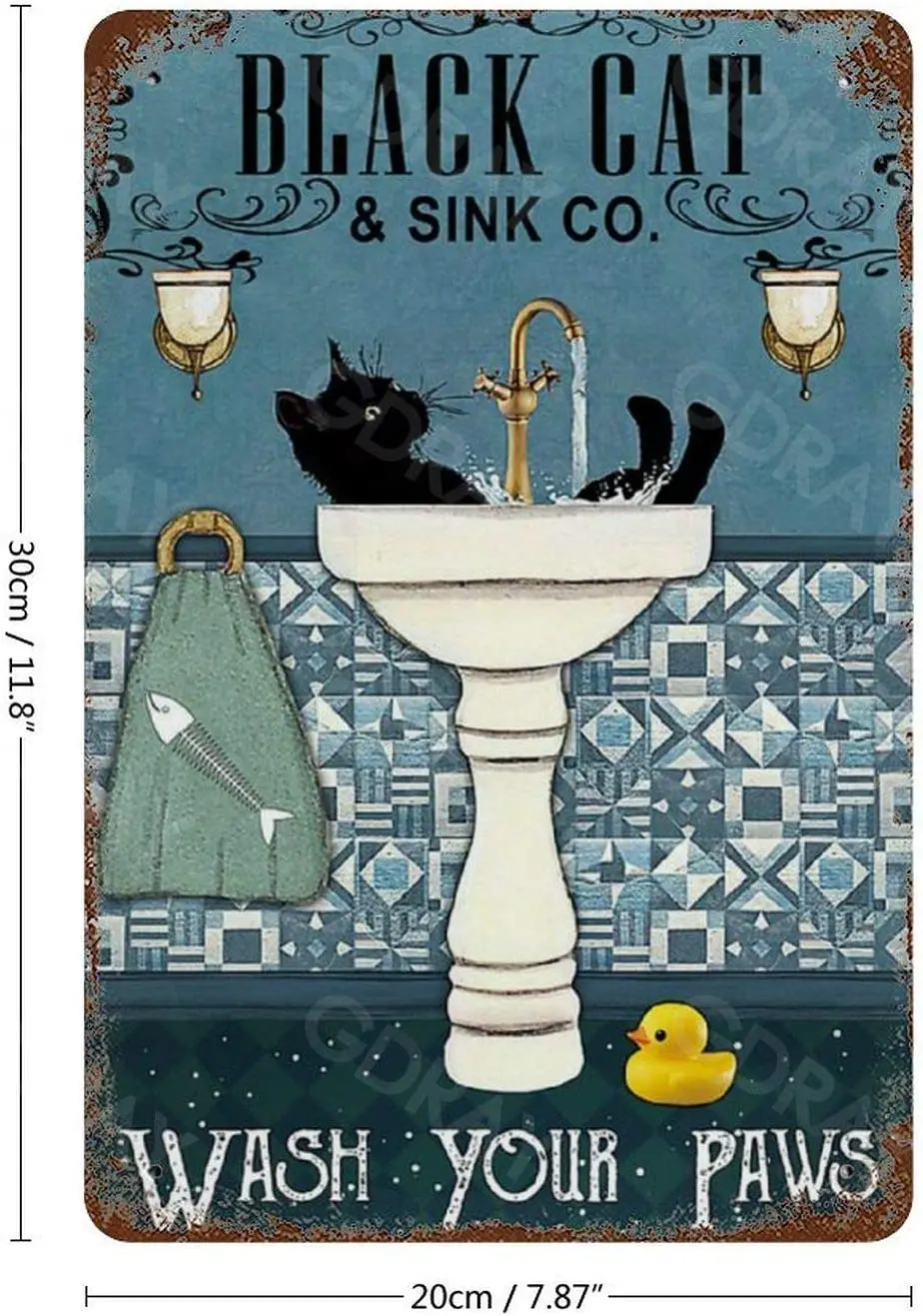This charming and whimsical printed plate sign is designed for bathroom decor. It measures 11.8 inches in height and 7.87 inches in width, and features a graceful rectangular shape with rounded edges. The sign bears the playful brand name "Black Cat and Sink Company" at the top in black font against a calming blue background. At the bottom, in an off-white font, it reads "Wash Your Paws."

The central illustration showcases an adorable black cat playfully situated inside an off-white pedestal sink. The sink is equipped with a golden brass faucet, out of which water is elegantly flowing. Flanking the sink are two wall sconces positioned symmetrically at the height of the faucet. To the left of the sink, there's a towel rack holding an aqua-green towel adorned with a fishbone design. Beneath the sink, on the right side of the pedestal, a cute little yellow rubber duck adds to the scene’s charm. The floor beneath the sink displays a mix of blue with hints of dark green, complementing the cozy, bathroom-friendly aesthetic of the entire piece.